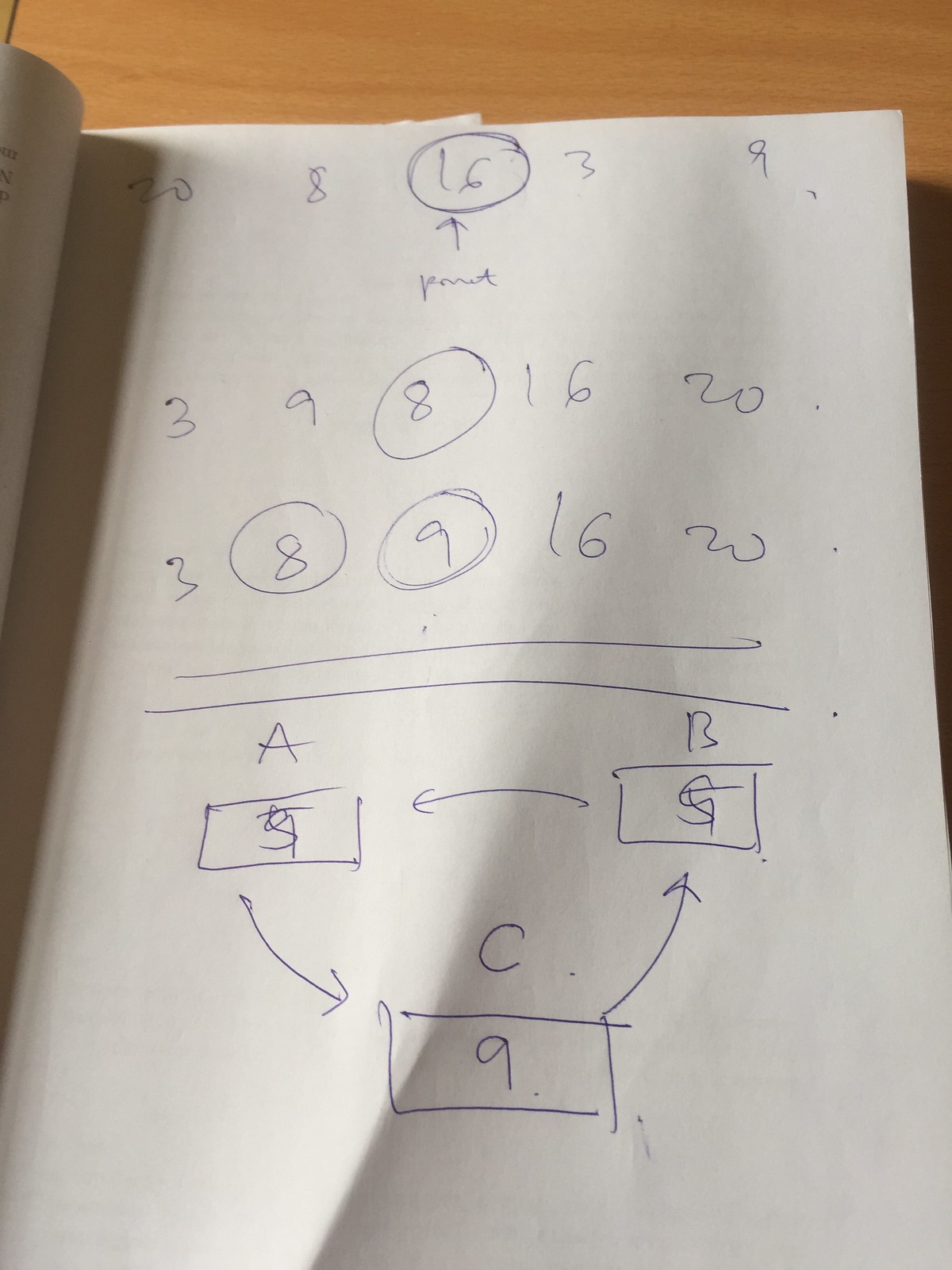A sheet of paper, predominantly occupying the photograph, lays on a wooden surface which is slightly visible at the top of the frame. At the apex of the page, written in blue pen, is the sequence "20 8 16," with the "16" enclosed in a circle. Following this, an illegible word with an accompanying arrow is inscribed, directing back to the circled "16." Proceeding the original row are the numbers "3 9" spaced out evenly. Below, the phrase containing the arrow and word is repeated.

Beneath this, another row lists the numbers: "3 9 8 (circled) 16 20." Following a similar format, yet another sequence is noted: "3 8 (circled) 9 (circled) 16 20," with this last row distinctly underlined twice.

At the bottom section of the paper are two large, labeled letters—'A' on the left and 'B' on the right. Below each letter, a rectangle is drawn. Further down and centrally aligned with the previous rectangles is another smaller rectangle, triangular in shape. Arrows curve around these rectangles, forming a circular flow diagram.

Within each rectangle, numbers are inscribed. The lower central rectangle distinctly displays the number "9." The upper two rectangles initially seem to have contained the number "9," but these have been overwritten with the number "5."